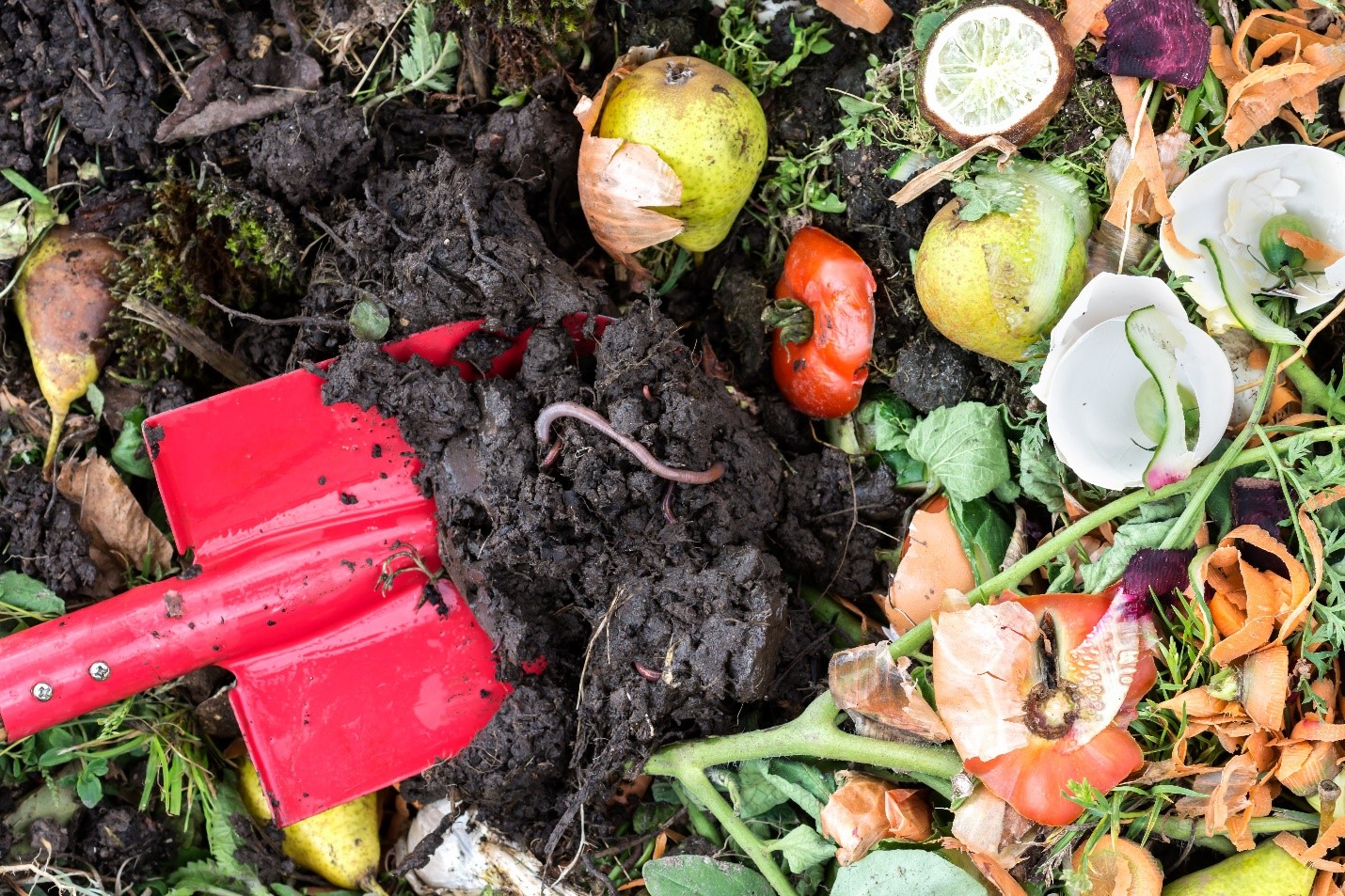In this close-up photograph of a compost pile, the rich, dark, muddy soil is prominently featured. At the left-hand side of the image, a red spade is partially buried in the soil, its handle out of view. The spade appears to be in the process of turning the compost, revealing an assortment of decomposing fruits and vegetables. 

Visible within the pile are a couple of pears, the remnants of tomato centers and stems, onion skins, carrot shavings, cucumber slices, some dried lemon or lime, and pieces of a bell pepper. Additionally, fragments of green plant stems and possibly some herbs are scattered throughout. A single pinkish-white earthworm is visible on the surface, further indicating the natural biodegradation taking place. 

Also noticeable are a few leaves and bits of grass interspersed within the compost, contributing to the overall assortment of garden and kitchen waste in the pile.